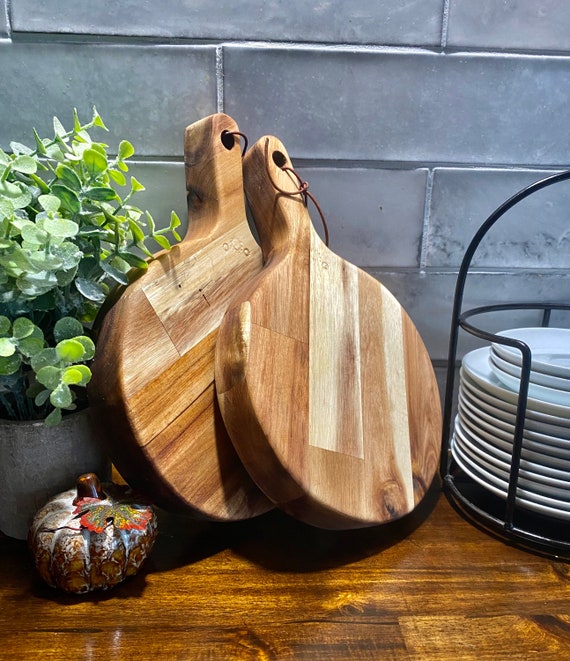In this photograph of a kitchen corner, a wooden countertop stretches across the frame with a cool gray subway tile backsplash setting a modern tone. On the left, a stone-like pot cradles a green plant with rubbery, eucalyptus-like leaves. Next to it sits a small, rustic decorative pumpkin in earthy hues with white detailing. Central to the scene are two round wooden cutting boards, their rich grain patterns and leather-stringed handles indicative of fine craftsmanship. The boards lean casually against the tile backdrop. To the right, a black metal plate rack holds a neat stack of white plates, adding a touch of practical elegance. This composition of elements – from the natural textures of wood and stone to the metallic and ceramic accents – creates a cozy yet stylish kitchen vignette.